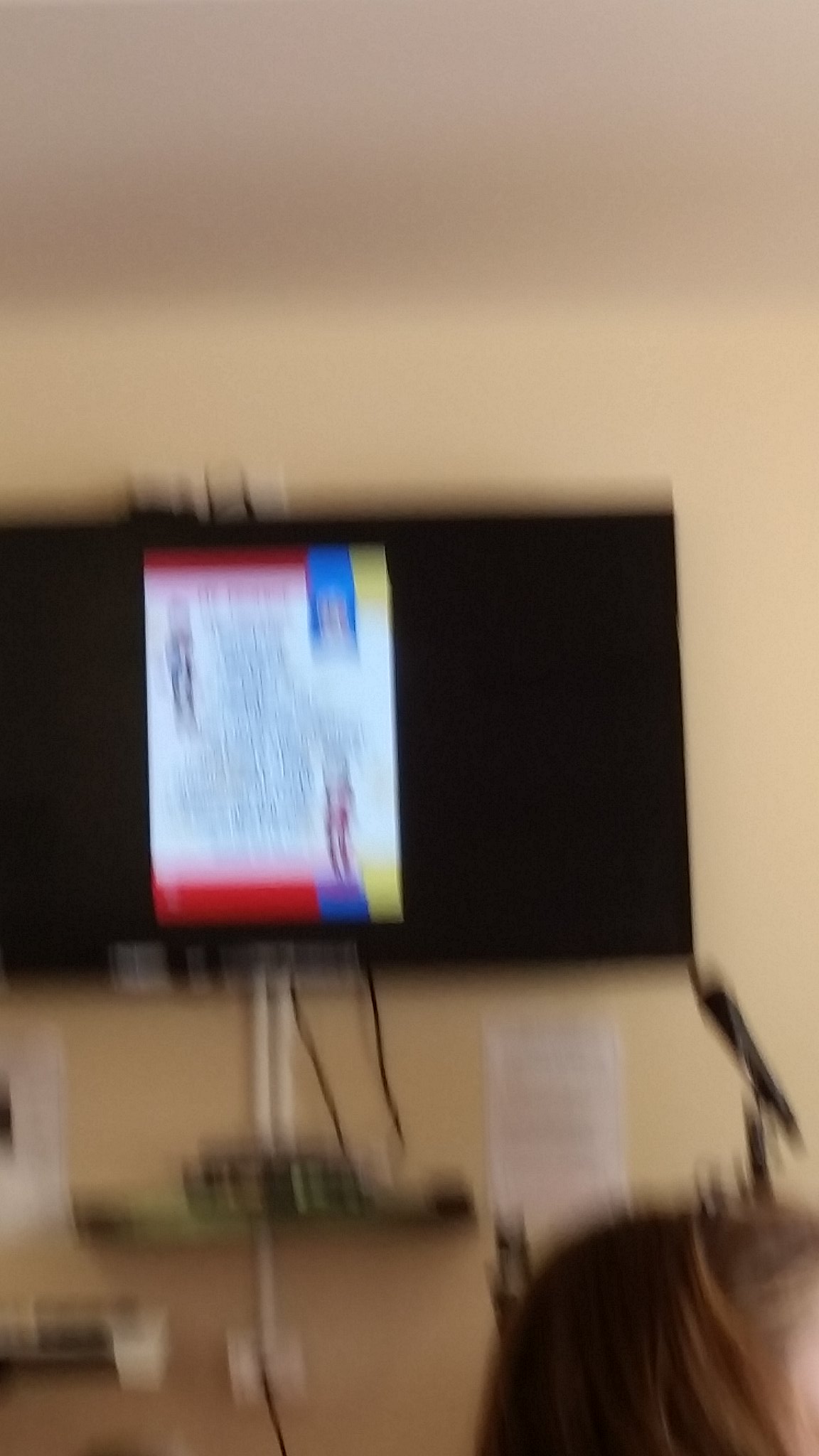This indoor color photograph, taken in portrait orientation with a smartphone camera, depicts a heavily blurred scene with distinctive elements suggesting it was captured in a public or educational space, such as a dormitory or lecture room. Dominating the center-left of the frame, a flat-screen TV is mounted on a yellow, possibly orange-ish, beige wall. Though the TV screen shows a predominantly white display with unreadable black text and decorative red, blue, and yellow stripes, the blur obstructs clarity. Several black cords trail down from the TV, leading into a receptacle on the wall and creating a slightly disorganized appearance. Below the TV, on both sides, two white A4 papers with illegible text are visible, seemingly notices taped or placed on the wall. In the bottom right corner of the image, the top of a female's head with straight brown hair is faintly discernible, adding a candid element to the scene. Shelving or a setup under the TV holds additional equipment, possibly a console, reinforcing the notion of this being a communal or functional space.